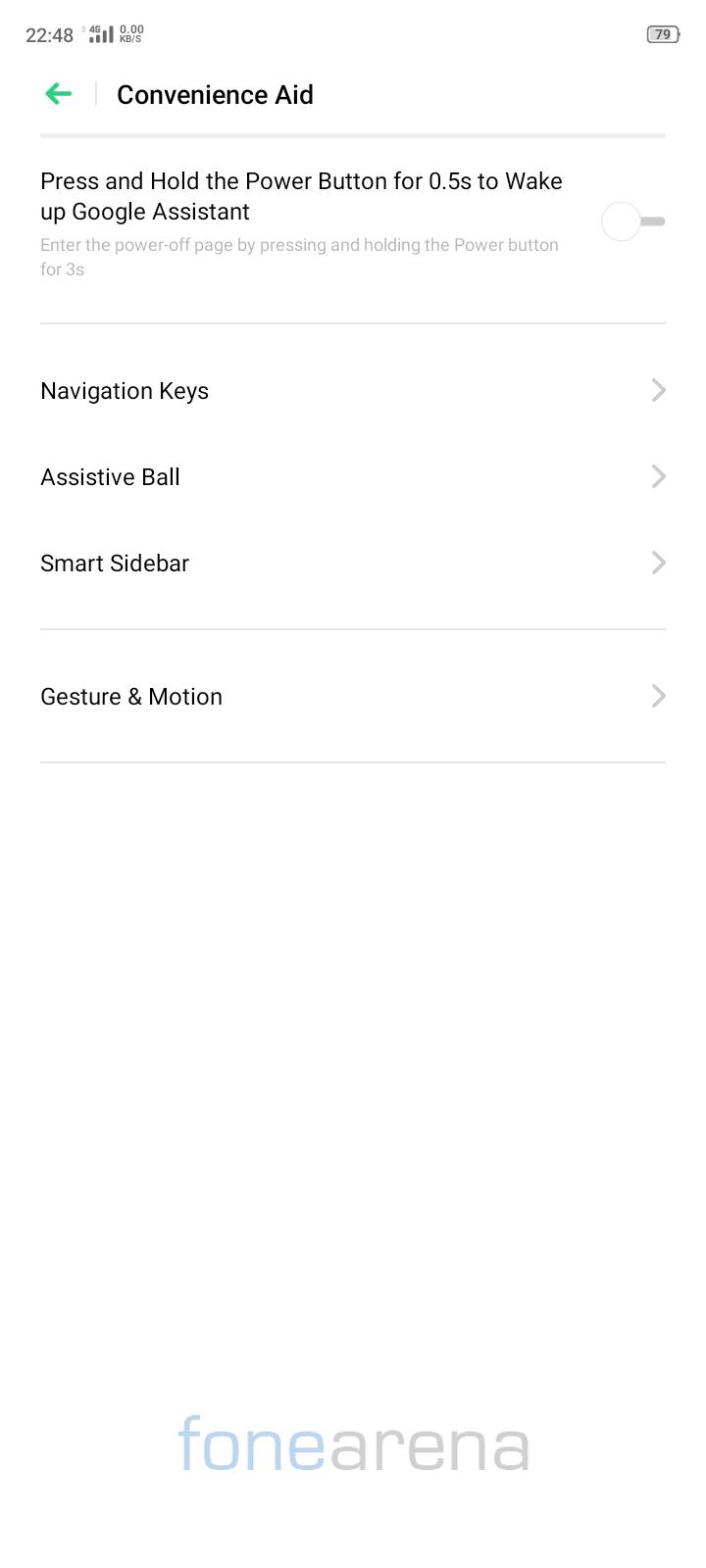This screenshot captures a minimalist interface from a cell phone, set against an all-white background. In the top left corner, the time is displayed in black as "22:48," accompanied by indicators showing a 4G connection with four bars, and a network activity status of "no KB/S." The upper right corner features a gray battery icon indicating "79" in black numbers. 

Below this, on the top left, a green back arrow is prominently visible. To its right, in large, bold black letters, the text "Convenience Aid" stands out. Underneath, a gray line separates the title from the instructions below, which read in black: "Press and hold the power button for five seconds to wake up Google Assistant." To the right of this instruction, there is a white toggle switch, currently set to the "off" position.

Further down, another gray line delineates this section. Below it, three options are listed on the left in black: "Navigation Keys," "Assistive Ball," and "Smart Sidebar," each accompanied by a gray right arrow on their respective far right.

At the very bottom of the page, framed by two gray lines, is the final entry, "Gesture and Motion," prominently displayed in bold black with a gray right arrow beside it. The footer of the screen features the words "phone arena" on the left in light blue font, and "fone arena" on the right in light gray font, with "fone" notably spelled as "F-O-N-E."